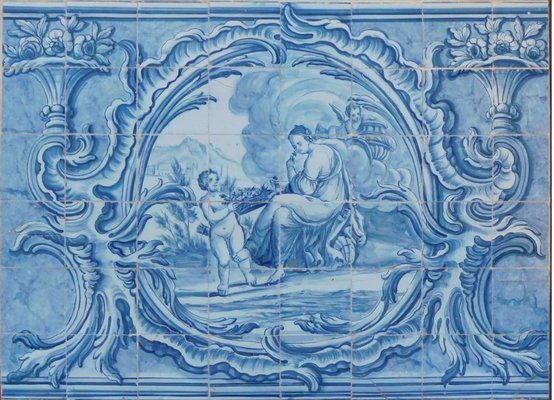This rectangular image, approximately three to four inches wide and three inches high, features a detailed blue tile mosaic. The individual tiles forming the mosaic are blue, with a very light blue grout in between. Each small tile varies in size, most being around half an inch to a quarter inch square. 

The central image, framed by a border resembling waves in a circular motion, depicts an outdoor scene reminiscent of the Greco-Roman period. At the heart of this scene is a woman seated with her legs crossed, adorned in a robe with her hair pulled up, evoking classical attire. In front of her, slightly to the left, stands a naked child holding what appears to be a basket of flowers, with a small quiver of arrows on their back, highlighting a cherubic presence. Another cherub is seen above the woman on the right, lounging on a cloud. 

The scene is encased in an elaborate frame, ending in decorative bouquets or stone sconces filled with flowers in the upper left and right corners. The background behind the woman includes the depiction of a tall mountain and a stone floor, adding depth to the portrayal of this serene and classical setting.